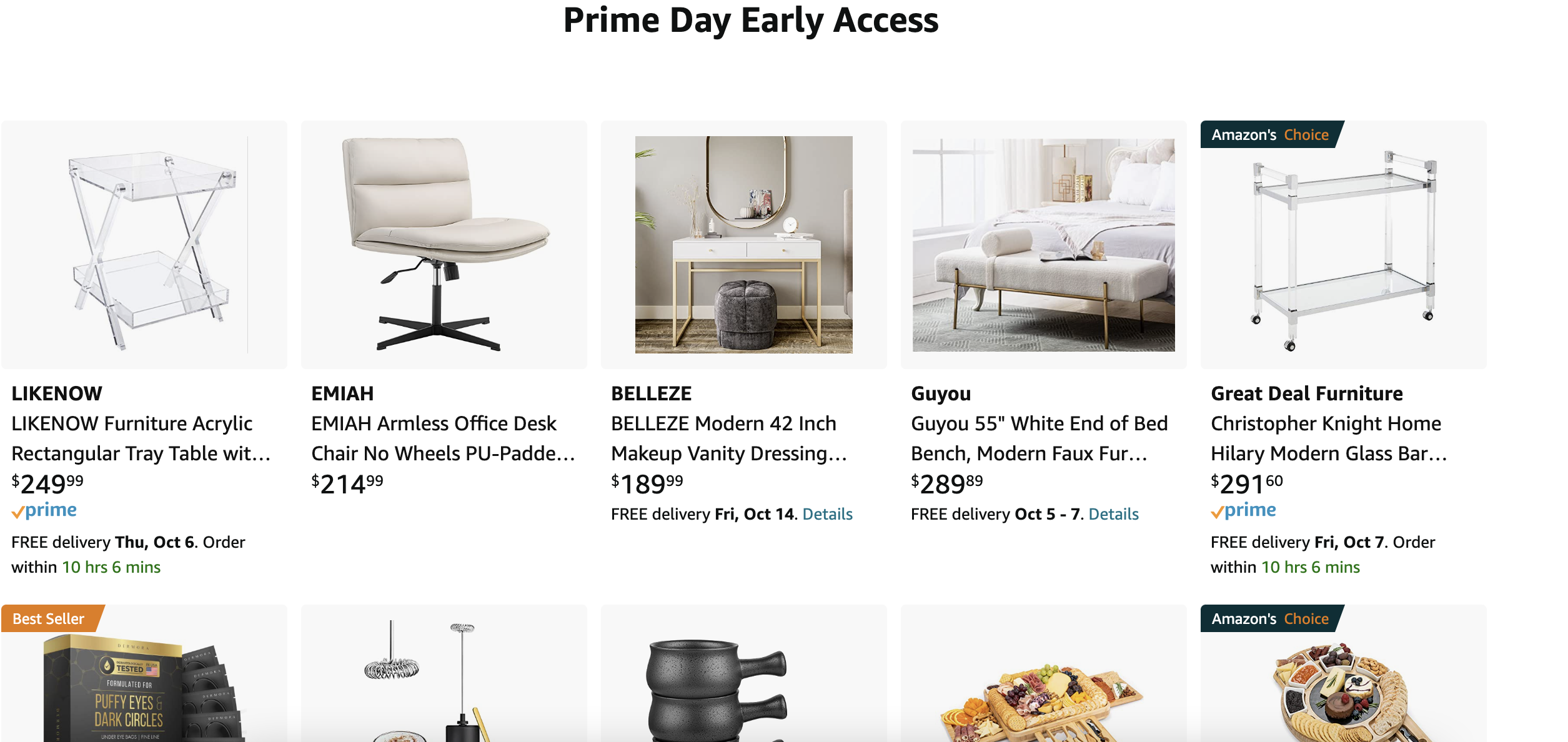The image showcases a selection of products available for sale with the "Prime Day Early Access" banner prominently displayed at the top in black text. Below the banner, five products are arranged from left to right, each with detailed information:

1. **Leichner Furniture Acrylic Rectangular Tray Table** - Priced at $249.99, this tray table features a sleek and modern design suitable for various settings.
2. **EMIAH Office Desk Chair** - This brand offers a light gray cushioned desk chair, priced at $214.99, promising comfort and ergonomic support.
3. **Belize Modern 42-Inch Makeup Vanity** - Available for $189.99, this vanity combines modern aesthetics with functionality for a sophisticated addition to any space.
4. **GoU 55-Inch White End of Bed Bench** - Priced at $289.99, this sturdy and stylish bench is perfect for adding extra seating or storage to your bedroom.
5. **Great Deal Furniture, Christopher Knight Home, Hillary Modern Glass Kitchen Rack** - This versatile kitchen rack is priced at $291.60 and offers elegant storage solutions with its modern glass design.

Each product listing includes a corresponding image and additional labels: the leftmost product is marked as a "Best Seller" (with an orange background and white text), while the product on the far right is labeled "Amazon's Choice" (with a black background; the first word in white, the second in orange). All products are set against a crisp white background, emphasizing their features and creating a clean, appealing visual presentation.